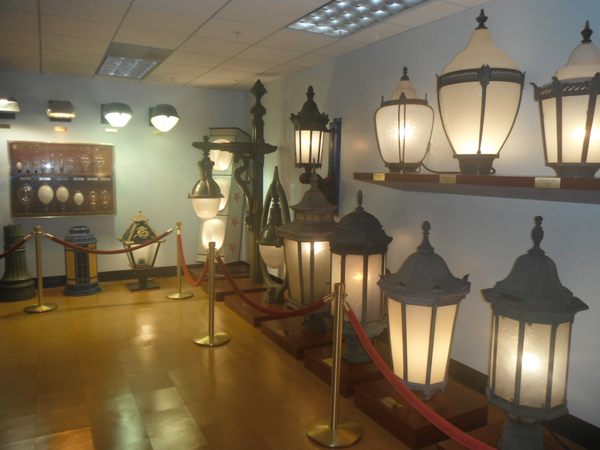The photograph depicts a museum exhibit dedicated to antique lanterns and light fixtures, enclosed by brass stanchions and red velvet ropes. The exhibit room features a shiny tan tile floor and white walls adorned with brown shelves. The shelves display a variety of ornate, Victorian-style lanterns with metal frames surrounding glass panels, many of which are illuminated. Along the left side, several lanterns rest independently on wooden boards. Towards the center, there is a single pole-mounted lantern, and to the right, four wall-mounted lanterns are displayed above a wall-mounted case showcasing various light bulbs. Additionally, larger light fixtures, possibly the upper parts of old streetlights, are placed on the floor, completing the intricate display of historical lighting devices. The ambiance is enhanced by four globe lights above the display case, likely providing necessary illumination rather than being part of the exhibit.